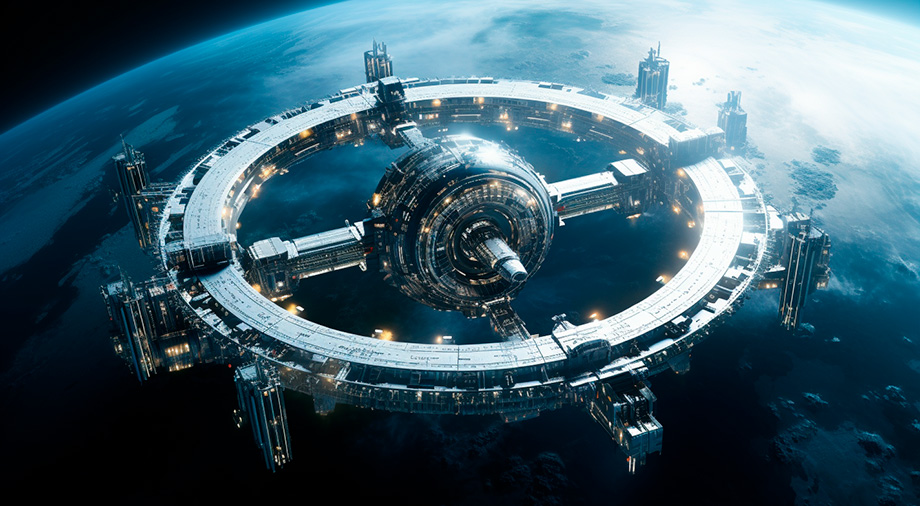This visually stunning, horizontally rectangular screenshot from a movie depicts a computer-generated image of an outer space scene featuring a circular space station prominently set against a vibrant interstellar backdrop. The primary object, a sleek, silver-toned space station, exhibits a complex and intricate design with interconnected hallways that intersect at a central spherical control area. The outer ring of the station is adorned with seven or eight structures resembling launch pads or docking stations for smaller crafts, reminiscent of metallic skyscrapers stretching into space. Illuminated with an array of lights, the space station gleams with modernity and futuristic allure. Beyond the station, a detailed view of a blue planet, potentially Earth, showcases visible landmasses, oceans, and swirling white clouds. The planet is bathed in sunlight, particularly noticeable in the upper right corner where a bright glare is present. In the upper left corner, the stark blackness of space serves as a contrasting backdrop, adding depth to this cosmic vista. The image, free of any text or figures, is vibrant and richly colored with a blend of blues, whites, and blacks, emphasizing the expansive and well-lit nature of the outer space setting.